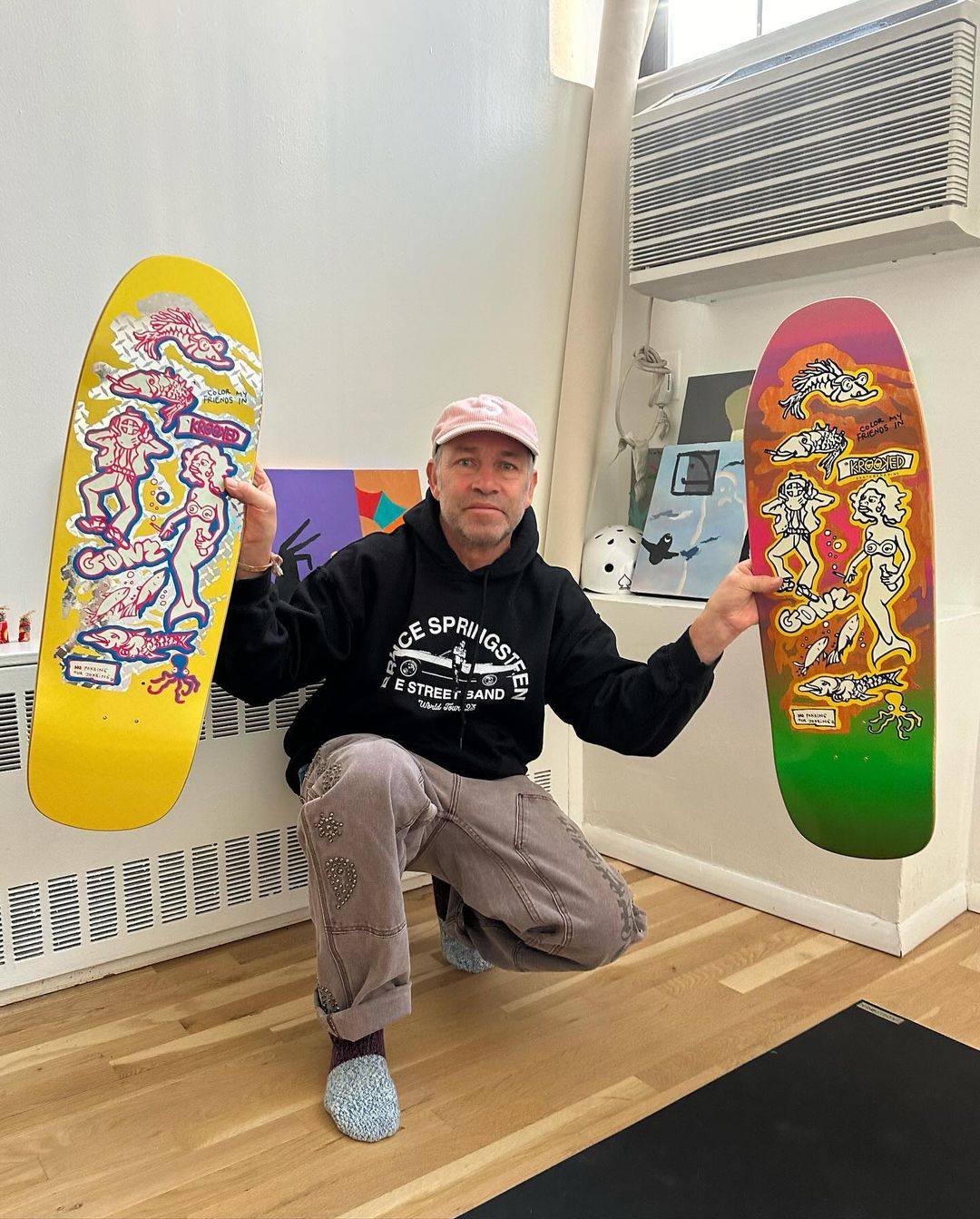A middle-aged man with gray hair and light stubble is posing in a room with gray walls and natural light streaming in from a window on the top right. The room features a wall AC unit and a tan floor. The man is wearing khaki pants, gray slippers (or possibly boat shoes), and a black hoodie with a Bruce Springsteen design. He has a pink hat partially covering his short hair.

In each of his extended arms, he holds a snowboard featuring artistic and colorful designs. The snowboard in his right hand has a vibrant yellow base with navy blue outlined drawings, including a mermaid, various fish, and a man wearing a diving helmet. The word "GONZ" is prominently displayed on this snowboard. In his left hand, he holds another snowboard with similar artistic designs, but on an orange and green base. The photo appears slightly compressed, affecting the image quality, and depicts the man kneeling or semi-kneeling on the floor.